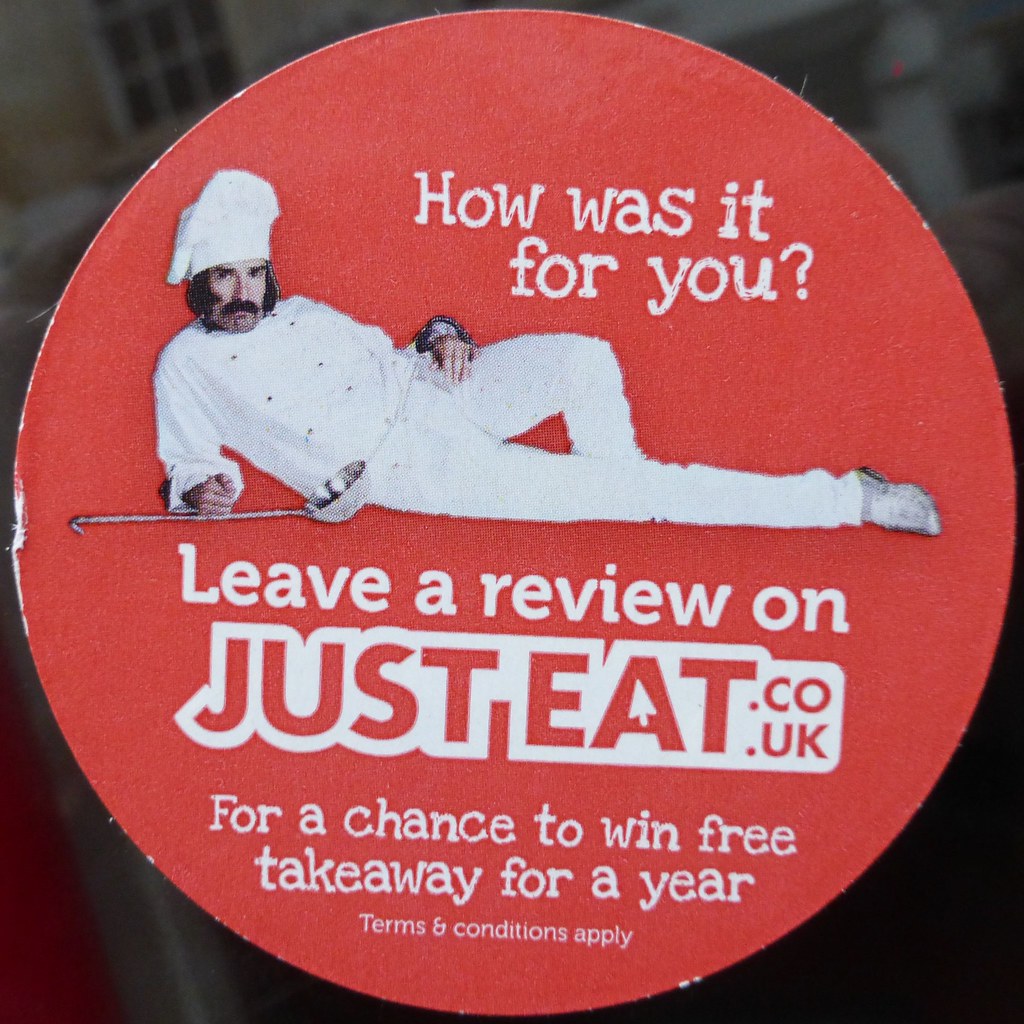The image features a distinctive red circle set against a black background, possibly part of another graphic with some white buildings visible. At the center, a chef is lying in a provocative pose, with one leg extended and the other bent, wearing a chef's hat and white uniform, including white shoes. He has short hair and a prominent mustache and is looking directly at the viewer. A large ladle rests on the ground beside him. Above him, in white text, is the question, "How was it for you?" and below that, "Leave us a review on justeat.co.uk" followed by "for a chance to win free takeaway for a year." The familiar Just Eat logo includes a unique detail: a computer mouse pointer embedded in the 'A'. Small text at the bottom indicates "terms and conditions apply," pointing to the promotional nature of the advertisement, encouraging customer feedback for a chance to win free meals.